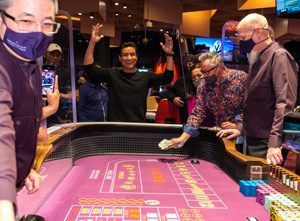In this slightly out-of-focus image captured during the pandemic, we see a bustling casino environment characterized by its high ceilings adorned with decorative panels and lighting. The centerpiece of the scene is a craps table, surrounded by players and bathed in the glow of nearby TV screens and video poker games. Most everyone is wearing face masks, indicative of the time. On the left, the dealer, wearing a dark blue face mask and glasses, leans towards the camera while reaching out with a device to draw back the dice. In the foreground, poker chips scatter across the right side of the table. At the end of the table, a man resembling Mario Lopez stands out in a black sweater, his sleeves pushed up, raising his arms in a triumphant pose with a broad smile, as if he's just made a winning throw. Nearby, an older bearded gentleman with white hair and another man with gray hair and dark glasses can be seen. One of them appears to be handling money on the table. The dynamic scene captures a moment of excitement and camaraderie under the constraints of pandemic protocols.